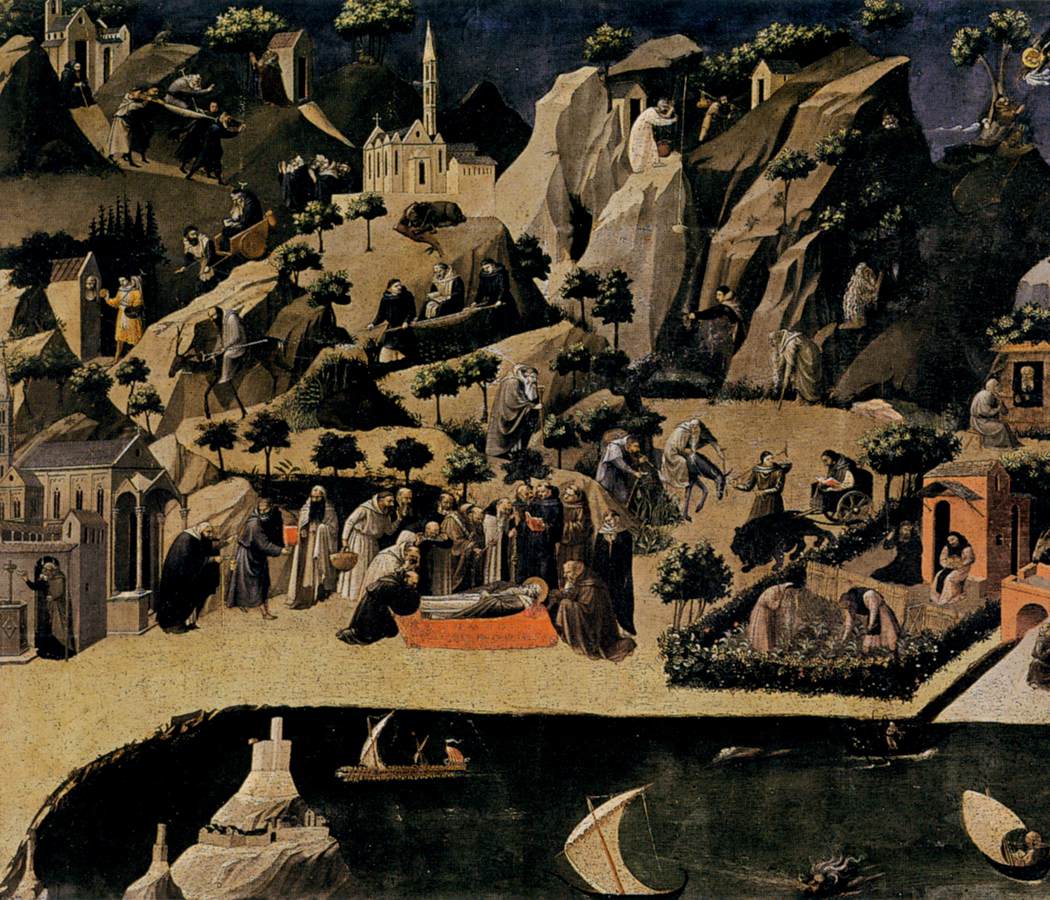This intricate painting, titled "Angelico," captures an ancient, biblical-like town built into a steep rock formation, painted in shades of brown, gray, and accented with melon orange. The town is below an eggplant-hued sky and visually tiered with layers of activity. In the foreground, there's a calm lake scattered with several boats, leading up to a bustling town square filled with people, mostly men. The townspeople are detailed in various activities: some are kneeling, some are standing, and to the right, a small group surrounds what appears to be a deceased person on a wooden platform, possibly praying.

Dominating the landscape on the left is a striking off-white church with a tall steeple, its entrance clearly visible. The church is surrounded by multiple residences and buildings. To the lower right of the church, there’s a figure resembling a man on horseback, and nearby a person in a wheelchair is visible. The rocky terrain varies in color from white to brown, with patches of bright yellow and other earthy tones, leading to more buildings and green-topped trees in the upper tiers. There are men pulling carts with women inside, adding a dynamic sense of daily life. Details like robes, baskets, and door-knocking figures contribute to the vibrant narrative of this historical scenery. The painting is rich in texture and color, offering a detailed glimpse into a town from ancient times.